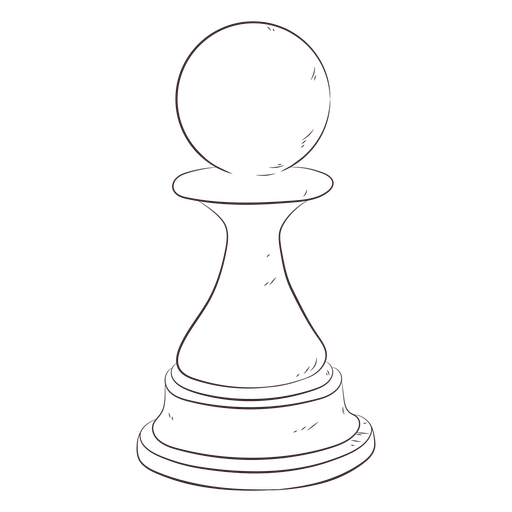This black-and-white image features a simple, hand-drawn line sketch of a chess pawn. The pawn, rendered on a white background, has a wide, solid base that tapers upwards into a rounded, beveled midsection, then narrows before flaring back out slightly. It is crowned by a solid, spherical top. Shadowy parts have been added to give the drawing a three-dimensional appearance. The entire chess piece dominates the picture, and the sketch lacks detailed intricacies or any other objects, making it a straightforward representation of a classic pawn, standing approximately three to three and a half inches tall and about two and a half inches wide.